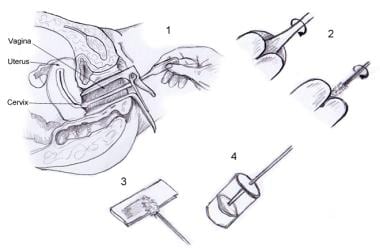The detailed diagram depicts a medical procedure involving the female reproductive system, focusing on the vagina, uterus, and cervix, which are all labeled. It contains four numbered illustrations, each highlighting a different step.

1. The first image in the upper left corner shows a cross-sectional view of the female reproductive system with a speculum inserted to open the vaginal canal. A hand is holding a long Q-tip, gently touching the cervix.
2. The second image in the upper right corner displays the same Q-tip moving in a circular motion on the cervix.
3. The third image in the bottom left corner demonstrates the end of the Q-tip being smeared onto a small piece of paper for sample collection.
4. The fourth image, located in the bottom right, shows the Q-tip being placed into a vial containing a liquid solution, presumably for preservation or further testing.

The diagram combines anatomical labels and procedural steps to clearly depict a method for collecting cervical samples.